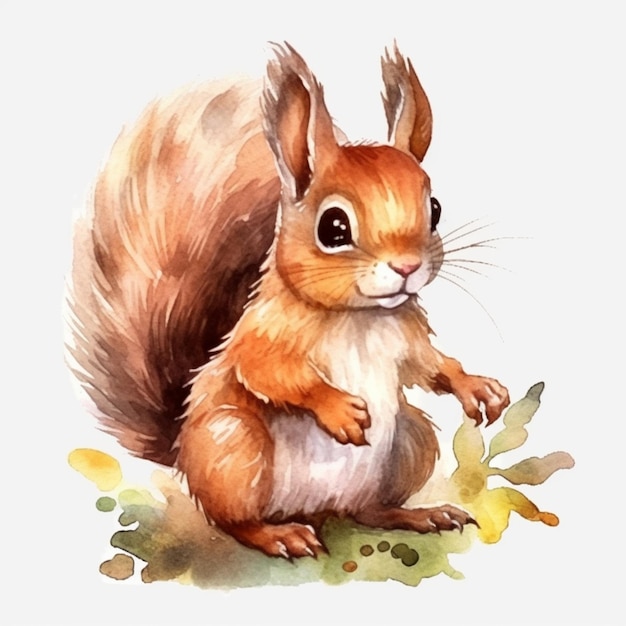This charming and whimsical children's illustration, created with watercolor or gouache, depicts an endearing baby squirrel. The squirrel, with its large, expressive brown eyes featuring a gleaming, cute sparkle, is facing slightly to the right. Its fur displays a palette of pinkish brown, light tan brown, dark brown, and gray, enhanced with meticulous highlighting and shading to provide texture and depth. 

The squirrel's distinctive large ears and bushy tail stand out, with the tail showing some darker shades of black towards the back. Sitting upright on its back paws, the squirrel's white belly is visible, and its short claws are detailed on both its front and back paws. It sits on a blend of green and yellow-toned foliage, suggesting a grassy or leafy environment, with a few red leaves and small nuggets scattered in front of it. The background of the painting is a very slightly off-white, allowing the vibrant colors and textures of the squirrel and foliage to stand out. The overall use of thick brush strokes adds texture and depth, enhancing the illustration's whimsical and attractive appeal for children.